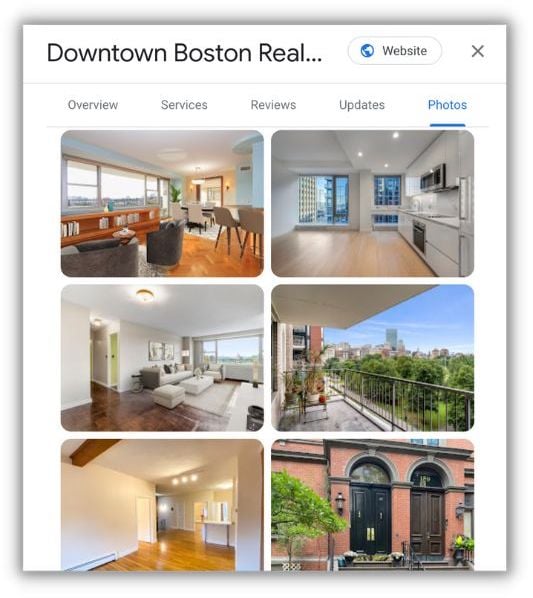This image captures a detailed webpage interface for Downtown Boston Realty. The main component is a white box framed by a subtle, shadowed gray border. Inside the box, the top section features the header "Downtown Boston Realty..." followed by a blue globe icon adjacent to a button labeled "Website." Next to it, on the right, is a small 'X' icon for closing the box. Below this is a navigation line listing the sections "Overview," "Services," "Reviews," "Updates," and "Photos."

The bottom section showcases a six-photo gallery. The top-left photo depicts a room with blue-painted walls, furnished with a table on a white rug and illuminated by expansive windows, with a view of hardwood flooring. Adjacent to this, the top-right image displays a kitchen with an empty counter and stove, also featuring hardwood floors but devoid of any additional furnishings. Directly beneath these, a photo captures a balcony scene overlooking a lush park, hinting at the serene and picturesque surroundings available in this urban environment.